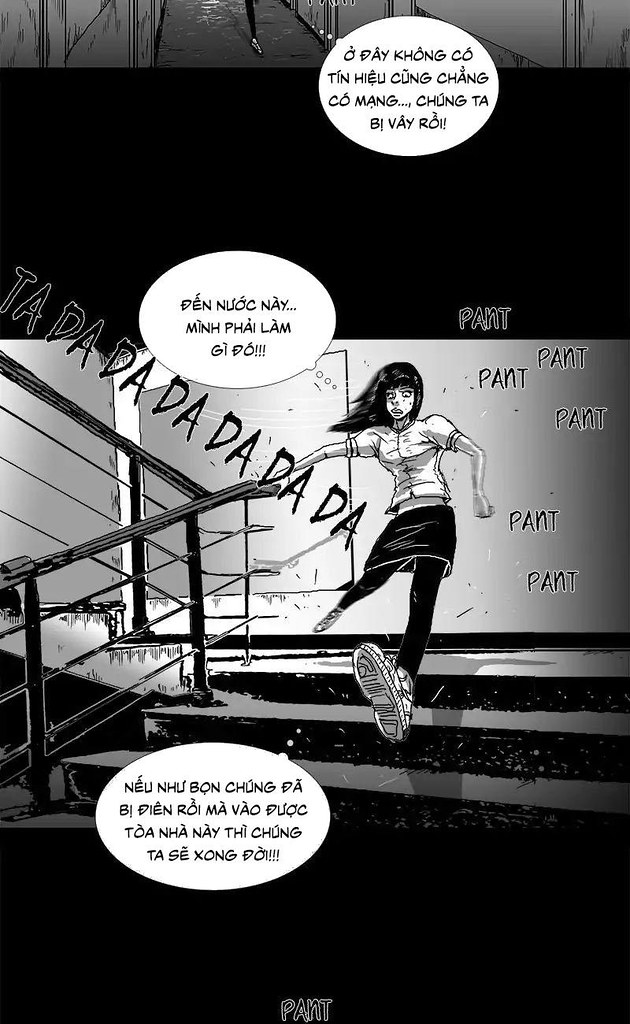This vertically oriented, black-and-white cartoon drawing appears to be a panel from a comic book. At the very top, part of an upper panel is visible, showing a figure likely walking in what seems like a hallway. This section features a speech bubble with text in an Asian language, possibly Chinese, Japanese, or another East Asian script. Below this, there is a black rectangle, followed by a panel illustrating a girl descending a staircase. The viewpoint is from below, providing a clear view of her extended foot stepping down.

The girl appears somewhat panicked or nervous, with text and speech bubbles surrounding her. As she moves, repetitive sound effect text, "ta-da, ta-da, da-da, da-da-da," follows the length of the handrail along the stairway, indicating the sounds of her footsteps. On the right-hand side of the image, more text spells out "pant, pant, pant, pant," illustrating her heavy breathing. Below her foot, another thought bubble is visible, adding to the sense of frantic movement. The overall composition and textual elements, including the detailed depiction of her stepping shoe and the clipped upper panel, convey a scene of hurried activity and anxiety.